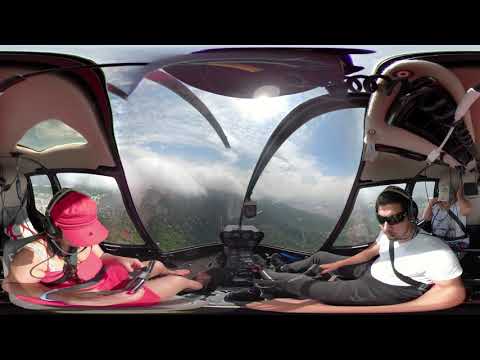In this detailed and immersive image, we are looking at the interior of a helicopter in flight, set against a stunning outdoor backdrop. The inside of the helicopter features a tan and possibly red interior, with various controls and devices visible in the central console. Seated in the front are two individuals. 

On the left, a woman dressed in a pink ensemble consisting of a cap, top, and skirt, dons a headset with a microphone and appears to be focused on a tablet or a similar device in her hand. Cables dangle around her neck area, emphasizing the advanced communication setup. Opposite her, on the right, is a man wearing a white t-shirt, dark pants, and black sunglasses. He also sports a headset and holds a control device in his right hand.

A third person is seated behind them, partially visible and wearing a white garment. This individual’s hands are raised above the heads of the two front passengers. All three occupants are securely strapped in with black seat belts.

Through the helicopter’s windshield, a breathtaking aerial view unfolds. The vibrant greenery below contrasts with a sky painted in hues of blue, dotted with fluffy white clouds. The sunlight pierces through, illuminating the scene. This image captures the essence of airborne adventure, blending the interior dynamics of helicopter flight with the stunning beauty of nature seen from above.